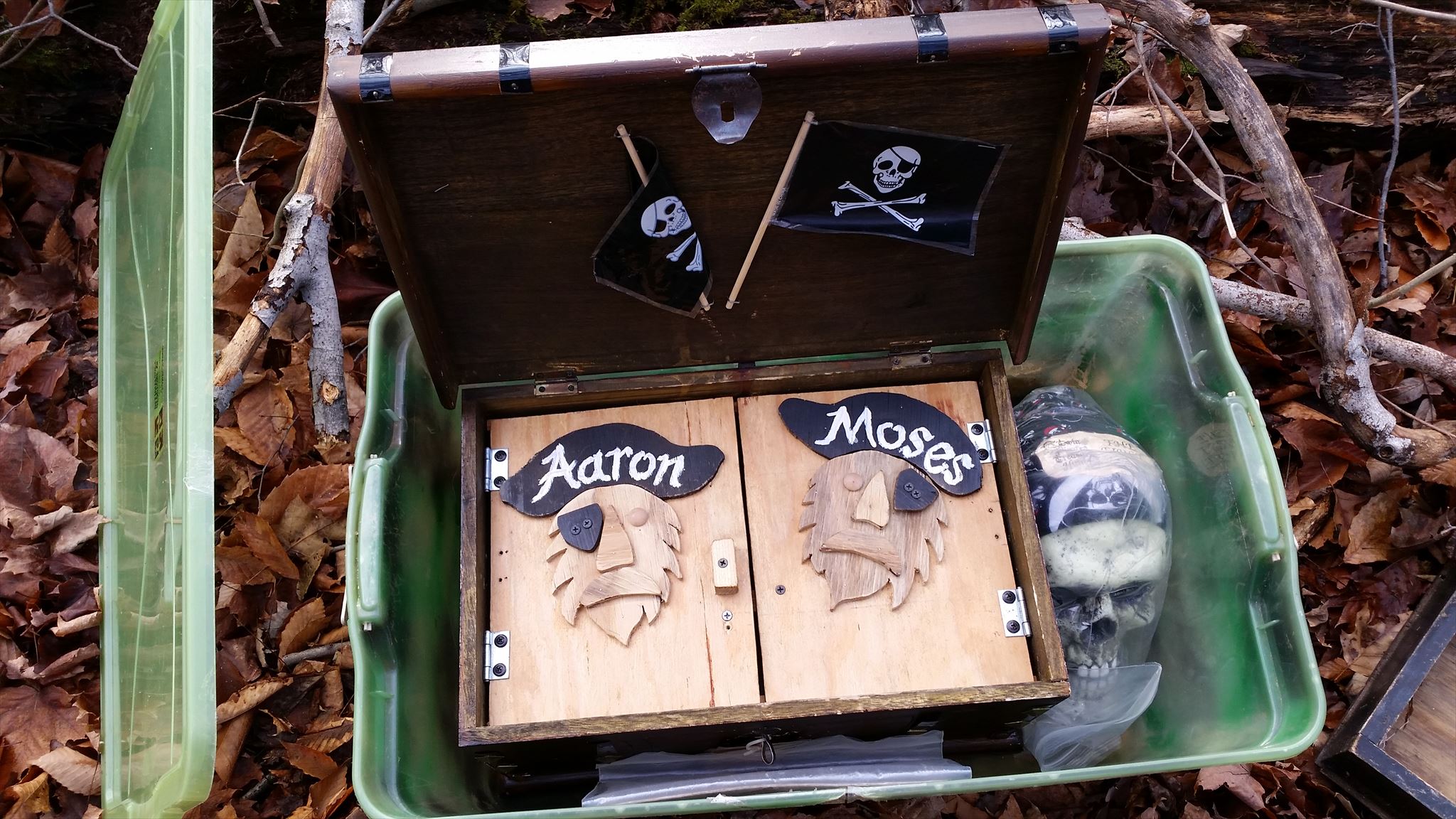The photograph depicts a large green transparent plastic tote outdoors, resting amidst a ground layer of dead leaves, stems, branches, and brush. The tote's lid is positioned vertically next to a nearby tree branch. Inside the tote, there is an open wooden trunk with silver hinges, featuring two rectangular wooden compartments topped with black pirate hats—one labeled "Aaron" and the other "Moses" in white lettering. Each pirate face has a black eyepatch. Two black pirate flags with white skull and crossbones adorn the inside of the trunk's lid. Also within the tote are documents encased in clear plastic bags and a human skull wrapped in plastic, resembling a Halloween decoration, lying on the right side. The entire scene evokes a sense of discovery, akin to finding a geocache treasure in the midst of nature.